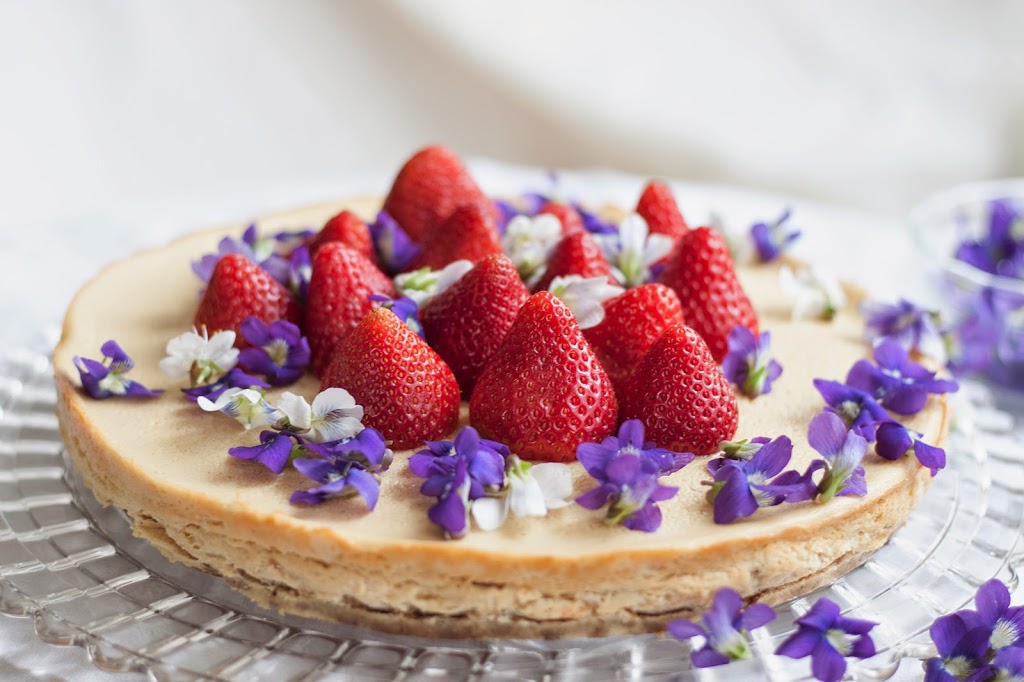This image showcases a flat, disc-shaped cheesecake tart adorned with approximately 15 vibrant red strawberries. Each strawberry's texture is clearly visible, adding to the visual appeal. Interspersed among the strawberries are delicate purple flowers with hints of white, elegantly decorating the tart’s surface. The tart itself rests on a clear, circular glass plate set against a plain white background, enhancing the vivid colors of the strawberries and flowers. The overall color palette of the image includes shades of red, purple, white, cream, and subtle hints of blue, creating a visually striking and appetizing presentation. No text is present within the image.